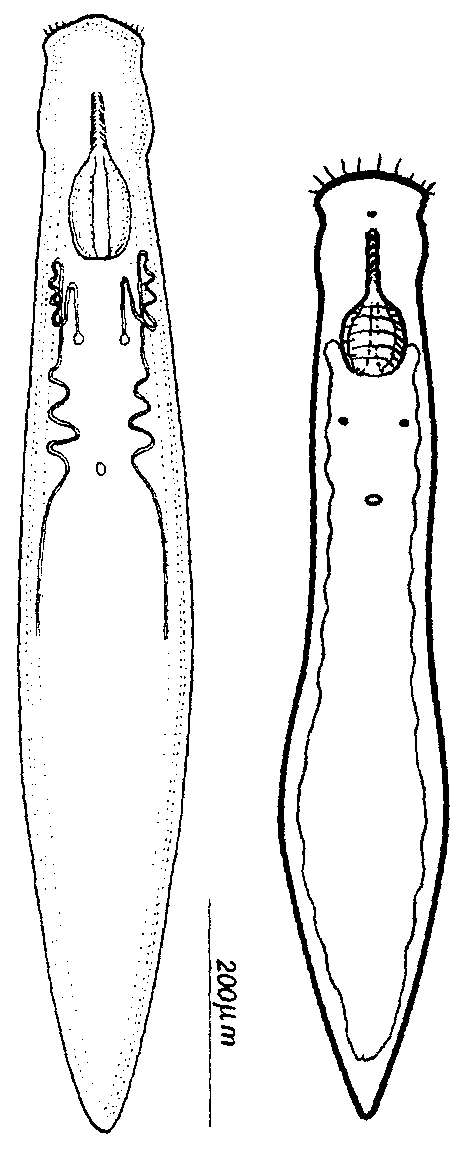The image depicts two detailed black and white design sketches displayed vertically, both slender and elongated with intricate internal structures visible. The sketch on the left is taller and spear-shaped, featuring a shape resembling a squash at the top, from which two wiggly lines extend outward on each side of a blank central area. This structure is complemented by visible lines and circles that accentuate its design. The sketch on the right, slightly shorter, also has a squash-shaped top that appears to resemble a llama's head with two eyes and a central circle. Both drawings have internal elements, such as organ-like lines and shapes, with the prominence of a vertical line marked "200 UM" denoting a measurement. The sketches, set against a white background, are meticulously rendered to display the structural intricacies and are devoid of any color, emphasizing the stark contrast and the elaborate details of their slender, worm-like forms.